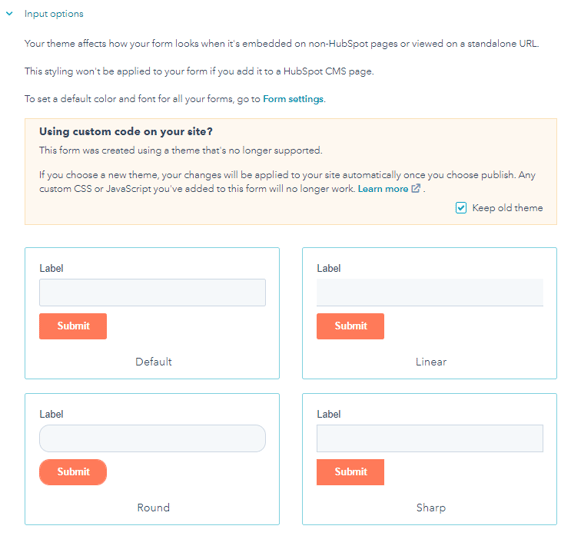The image depicts a page from an unspecified website. The page lacks a URL bar, making identification of the website impossible. 

At the top left corner, in bold blue text, the page header reads "Input Options," accompanied by a blue down arrow. Directly below this header, there is an informative line in black text: "Your theme affects how your form looks when it's embedded on non-hotspot pages or viewed in a standalone URL."

Beneath this text block, there's a broad rectangular area with a cream-colored background. In the top left corner of this section, a bold caption states, "Using custom code on your site?" Followed by a smaller informational text: "This form was created using a theme that's no longer supported. If you choose a new theme, your changes will be applied to your site automatically." 

In the bottom right corner of this cream section, there's a "Learn more" link in blue text, next to which is a small gray square icon featuring an up arrow. Additionally, at the very bottom right, a blue outlined square encloses a blue check mark with the label "Keep old theme."

Below this cream section, there are two rows, each containing two blue-outlined rectangular sections meant for user inputs. Each input area is labeled in black text in the upper left corner with the word "Label." Under each label, there is a gray-outlined entry bar. Accompanying each entry bar on the left is a red rectangular button with white text reading "Submit."

The final distinction between these sections is marked at the center bottom of each box with black text: 
- The top left box is labeled "Default."
- The top right box is labeled "Linear."
- The bottom left box is labeled "Round."
- The bottom right box is labeled "Sharp."